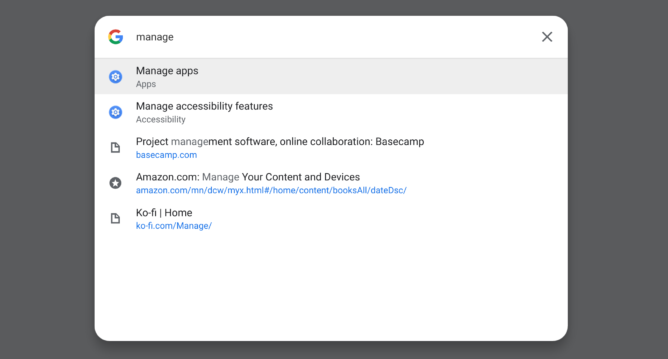This image showcases the settings or management section for Google, featuring a clean, minimalist design. The background is a solid dark gray color that provides a sleek and modern aesthetic. Prominently displayed in the center of the image is a white rectangular tile with rounded corners, drawing immediate attention.

At the top of this tile, on the left-hand side, is the recognizable Google logo, conveying the brand's identity. Positioned to the right of the logo is the word "Manage," guiding users on the purpose of this interface. In the upper right corner, there's a black 'X,' likely serving as a close or exit button for this settings window.

Directly under this header, a section titled "Manage Apps" is highlighted with a blue icon to its left, indicating its functionality. Below, another section is labeled "Manage Accessibility Features," also marked with a different blue icon to signify its unique purpose.

Continuing down the tile, there's a segment that features an icon resembling a piece of paper. This section is labeled "Project Management Software: Online Collaboration Basecamp," suggesting tools for project management and collaboration. Beneath this, a star icon leads into a section titled "amazon.com: Manage Your Content and Devices," which appears to link to Amazon’s management interface for user content and devices. Finally, another paper icon introduces the section "Ko-fi: Ko-fi Home," likely relating to the Ko-fi platform for supporting creators.

Overall, this well-organized and visually appealing management section offers a clear and intuitive user experience for accessing various settings and management features.